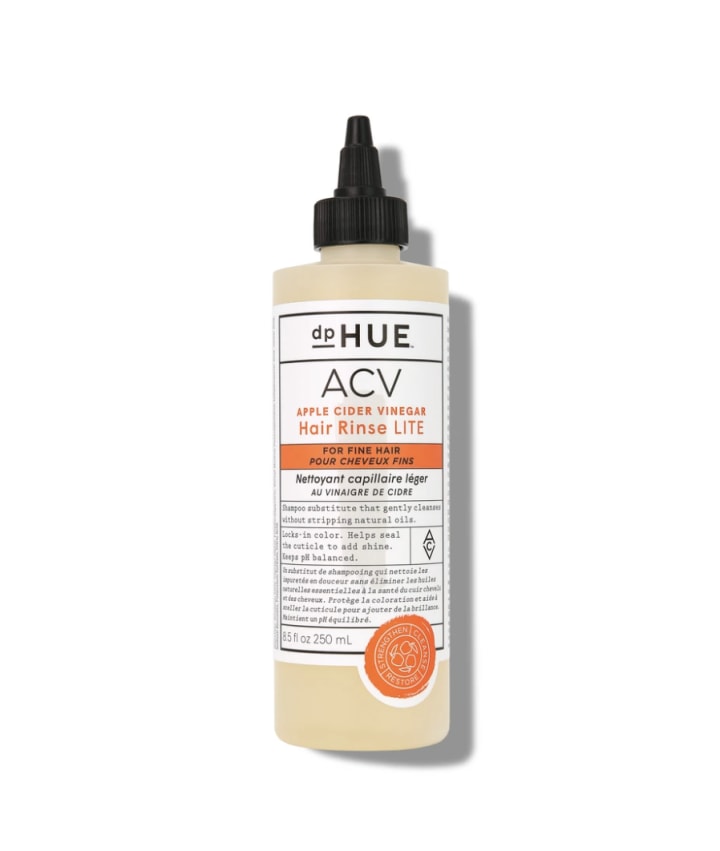The image features a long, cylindrical plastic bottle with a black, conical cap that has a rough, outer grid pattern for easy grip. The bottle is a creamy beige color and is adorned with a white label that has a black border. In the center of the label, there's an orange text bar and an orange stamp logo in the bottom right corner, with a wax-seal appearance. The black text on the white label reads "D.P. HUE," while the orange text specifies "Apple Cider Vinegar Hair Rinse, Light." Below this, the orange text box with black writing states, "For Fine Hair," followed by a passage likely in another language: "Pour chavoux fin, nettoyant capillaire lagar, en vinaigre de cidre." Additional text boxes below contain paragraphs of ingredients and warning labels, some possibly in different languages. This entire setup rests on a plain white background.